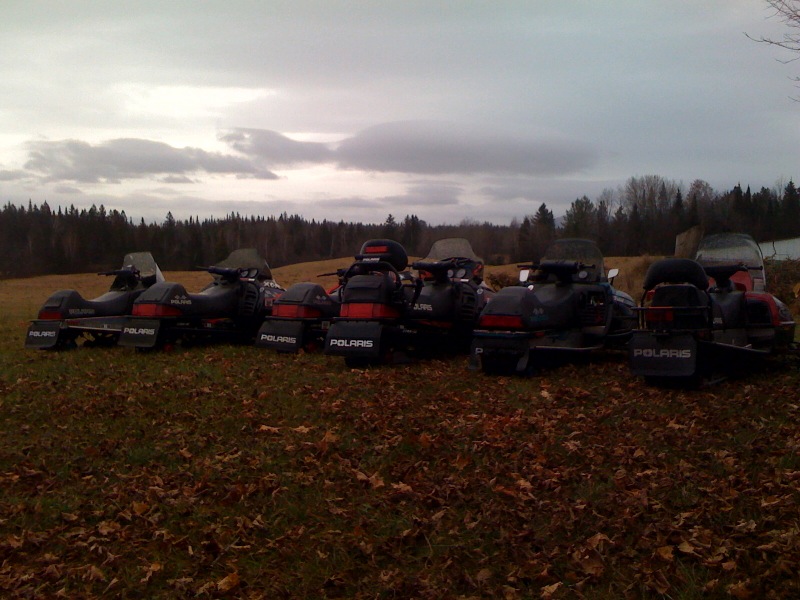This color photograph captures a row of Polaris snowmobiles parked on a dark grassy field with numerous dead leaves scattered in the foreground. The sky above is overcast with clouds, casting a dim, evening light over the scene. In the distance, we can observe a lush meadow bordered by tall pine trees, creating a serene natural backdrop. The snowmobiles are aligned in such a way that we are looking at their backs, allowing a clear view of details such as the rear flaps, backlights, and seats. Despite the dim lighting, the instrument panels and windshields facing away from the viewer are visible. No other writing or signage appears in the photograph, which is devoid of people, animals, or buildings. The right side of the image is particularly dark, making it challenging to count the exact number of snowmobiles, though there appear to be at least eight. Overall, the scene combines the rugged functionality of the snowmobiles with the tranquil beauty of the natural setting.